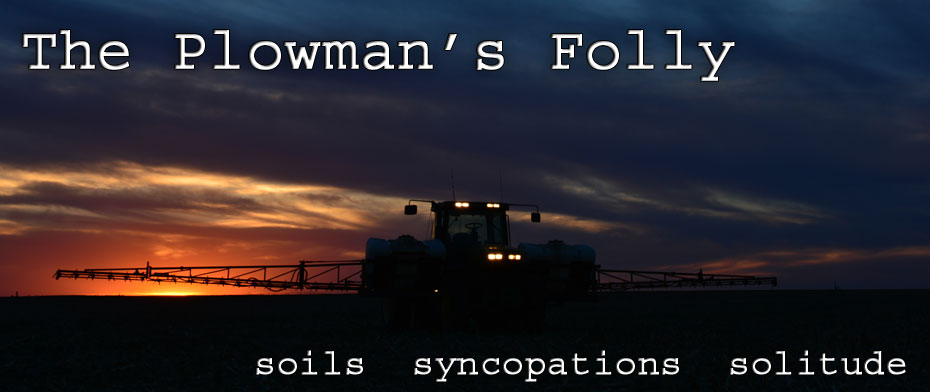A photograph captures a dusk scene with a combine tractor equipped with bright lights, operating in a field. The sky is painted with dramatic hues of dark blue and orange as the sun nearly slips below the horizon, casting a gloomy, cloud-covered atmosphere. Bold white lettering spans across the top left of the image, proclaiming “The Plowman’s Folly” in uppercase letters. Towards the lower right, smaller white text lists “soils, syncopations, solitude” in a more understated lowercase font. The dark lighting obscures the exact work the tractor is performing, but it highlights the solemn and solitary nature of farming at twilight.